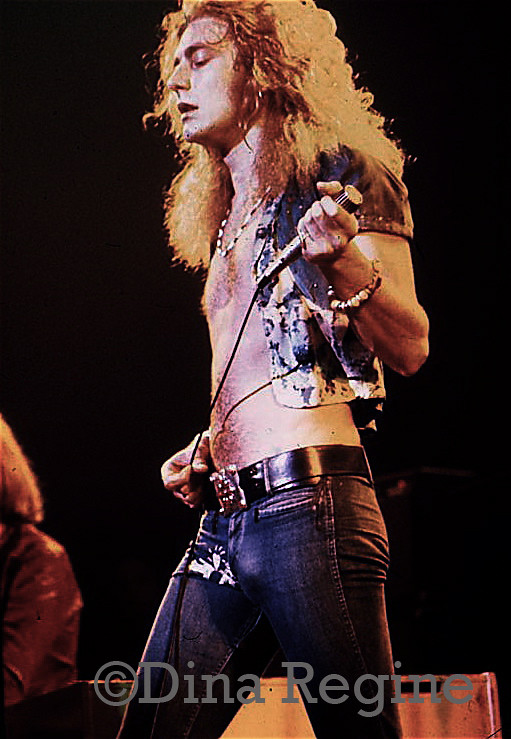The image captures the iconic lead singer of Led Zeppelin in the midst of an electrifying stage performance, likely from the late 70s or early 80s. He stands in a casual, yet powerful stance with one leg forward and the other back, embodying the raw energy of rock. His long, blonde, wavy hair flows freely as his eyes remain closed, lost in the music. He grips a microphone with his right hand, adding to the dynamic scene. His attire includes a sparkling, silvery jacket left open to reveal his bare chest adorned with visible chest and stomach hair. He accessorizes with a beaded necklace and a bracelet on his left wrist. His tight blue jeans, cinched with a black leather belt featuring a silver buckle, complete his quintessential rock star look. The bottom of the image carries a copyright mark "© Dina Regine" in gray. To his left, partially visible, is another performer in a red jacket with shoulder-length blonde hair, adding depth to the scene.